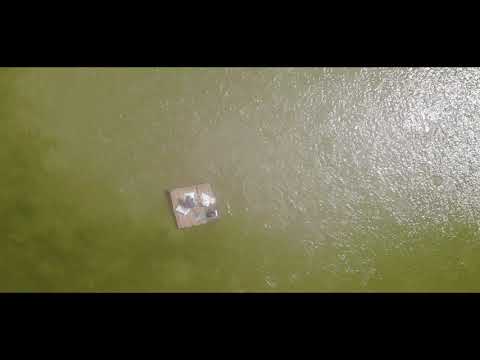This image, an outdoor, aerial photograph taken during the day, features a broad expanse of greenish, brownish water rippling with waves. The water, reflecting sunlight on the right side, brightens towards that area. Near the bottom left center of the image floats a square, brownish object, potentially a raft or some floating debris. This object, with some white splotches and a darker area, might be carrying unidentified items. The scene is slightly blurry and the photograph, in landscape orientation, is centered within a horizontal black strip at the top and bottom, enhancing its realistic, representational style.